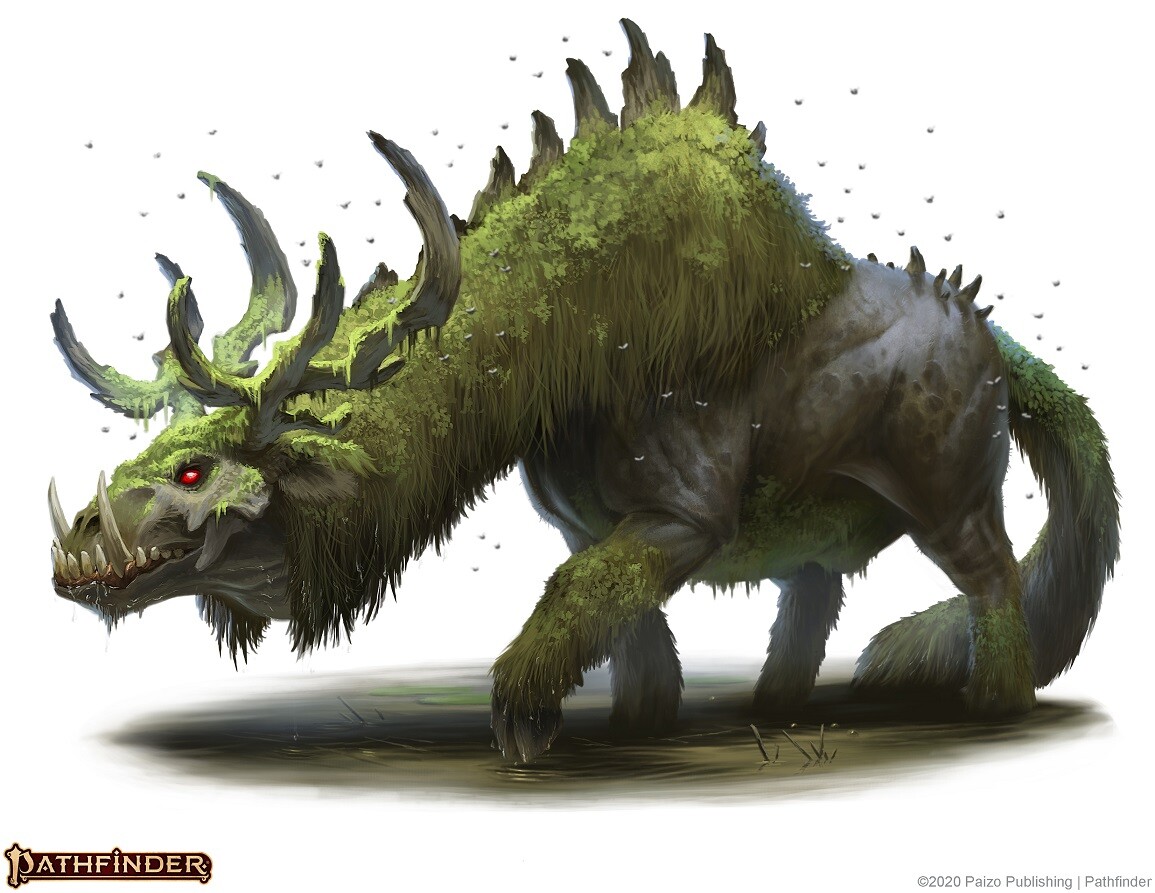This is a detailed digital illustration of a fantastical creature from the video game Pathfinder. The image prominently features the Pathfinder logo in the bottom left corner. The creature depicted is an intriguing mix of various animals, resembling a hybrid of a tiger, dog, cat, and giraffe with a notably long neck. Its head is adorned with antlers, and it possesses a pronounced, elongated bottom jaw filled with upward-pointing snagged teeth. The creature's eyes are a striking red, adding to its menacing appearance.

Its body is covered in what appears to be a mixture of fur and scales, with the fur resembling moss and other plant life, giving it an almost symbiotic relationship with nature. Along its spine and back, the creature has scales that resemble the pointed, rugged ridges of a stegosaurus, enhancing its prehistoric and fierce aesthetic. Surrounding the creature are what appear to be small bugs or birds, adding an element of liveliness to the scene.

The entire background is a clean white, emphasizing the detailed and abstract nature of the creature. The image highlights the creature’s unique blend of features, making it a compelling and imaginative addition to the world of Pathfinder.